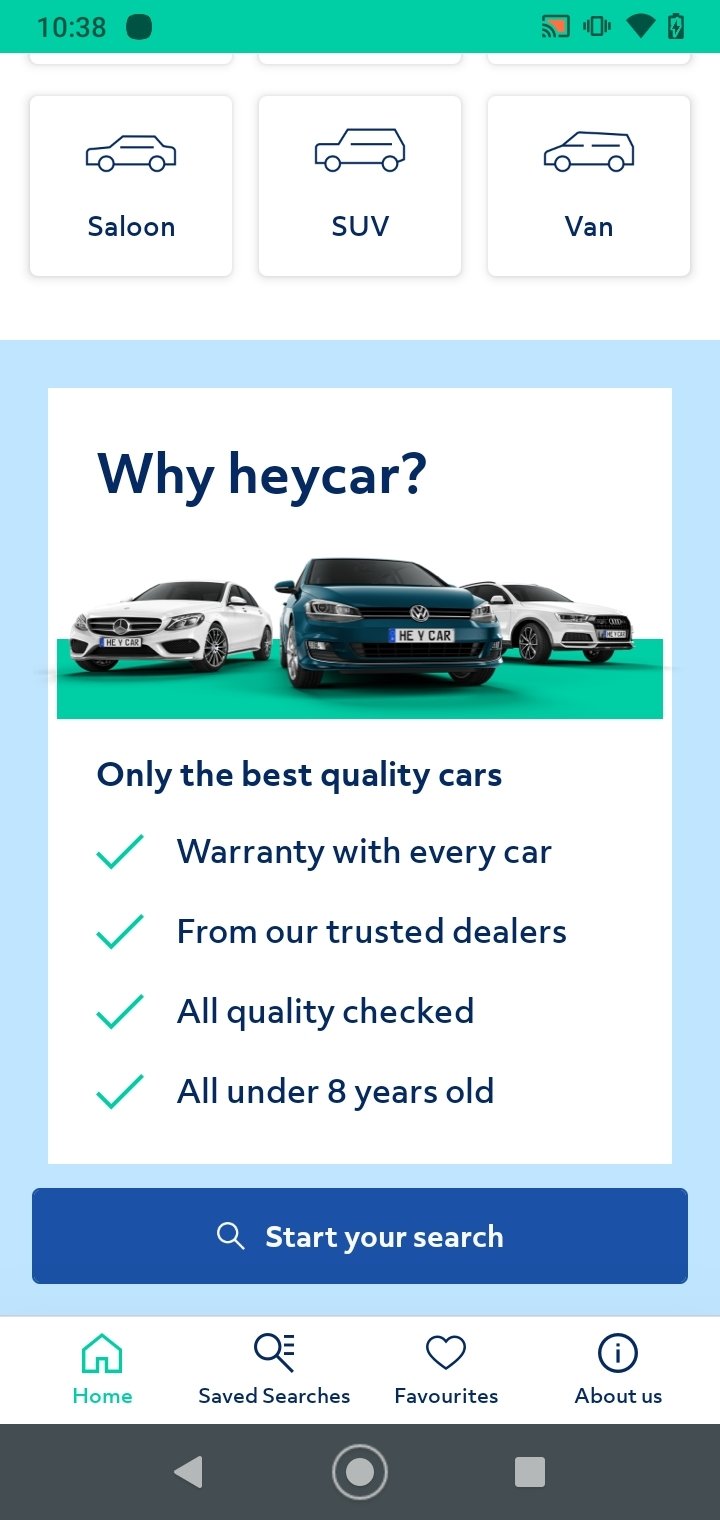**Detailed Screenshot Description:**

The image is a screenshot captured at 10:38, clearly showing the current time. The battery life indicator is alarmingly low, hinting at the need for a recharge soon. Additionally, the signal strength appears subpar. These elements are all encapsulated within a green status bar at the top of the screen.

Beneath the status bar, the main content of the screenshot is displayed against a white background. This section prominently features images of various types of vehicles including a sedan, an SUV, and a van, each accompanied by an illustrative drawing. 

A striking blue box bears the question, "Why a car?" followed by a series of selling points about the vehicles: "Only the best quality cars," "Warranty with every car from our trusted dealers," "Air quality checked," and "All under eight years old."

Just below these points, three cars are showcased, one of which is a Mercedes. The Mercedes features a playful license plate that reads, "Hey, car."

Further down, a dark blue call-to-action box invites users to "Start your search." 

At the bottom of the screen, a green section houses navigation options with icons: "Home," "Saved searches," "Favorites," and "About us." Finally, the very bottom of the screenshot contains navigation buttons including a left-pointing arrow, a home button, and a close button.